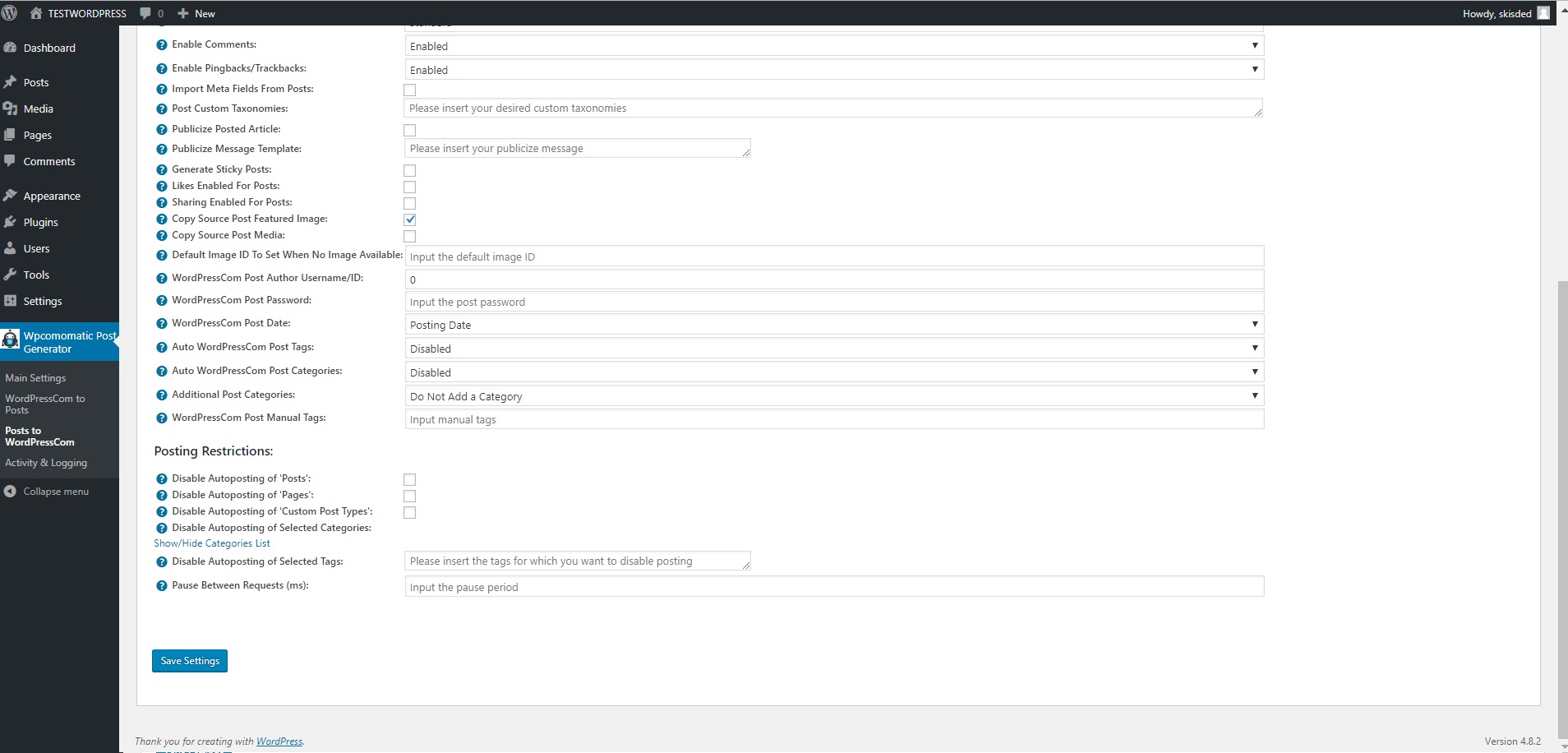This image showcases a WordPress dashboard screen, specifically a test environment for managing WordPress settings. On the left side, the recognizable "W" logo signifies WordPress. The menu reveals no comments are currently indicated, and a notification or option labeled "New" is present.

The left sidebar, shaded in black, displays a vertical menu that includes the following options: Dashboard, Posts, Media, Pages, Comments, Appearance, Plugins, Users, Tools, and Settings. Among these, "WP Comatic Past Generator" is highlighted in blue, indicating it is the selected section.

Further options are displayed in plain text, including Main Settings and WordPress.com to Posts. Highlighted in white is the section titled "Posts to WordPress.com," followed by Activity and Logging. There is also an option to collapse the menu for a more streamlined view.

Within the settings area, users have the option to enable comments and other features. Scrolling down, there is a section dedicated to posting restrictions, such as disabling the auto-posting of posts. At the bottom of this screen, a "Save Settings" button is available for users to apply any changes made. This interface appears to be designed for comprehensive control over WordPress functionalities.